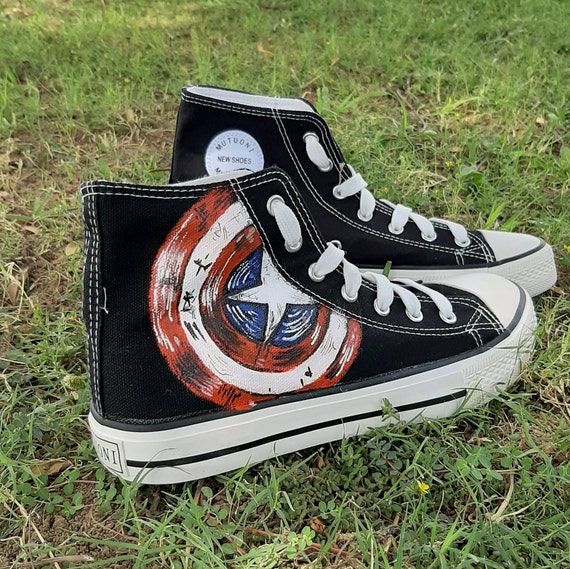This color photograph features a pair of high-top sneakers, resembling Converse, sitting on patchy grass. Both shoes have black canvas uppers with white stitching, silver grommets, and white laces. The soles and toe caps are made of white rubber with a black stripe running along the soles. The right shoe, prominently in the foreground, displays a painted Captain America shield on its inner side, featuring a blue center with a white star, surrounded by alternating red and white rings. The left shoe, visible in the background, has a white circular logo on its outer side, reading "Mutoni New Shoes." Both shoes are positioned with their toes pointing towards the right side of the image, creating a slightly slanted arrangement.